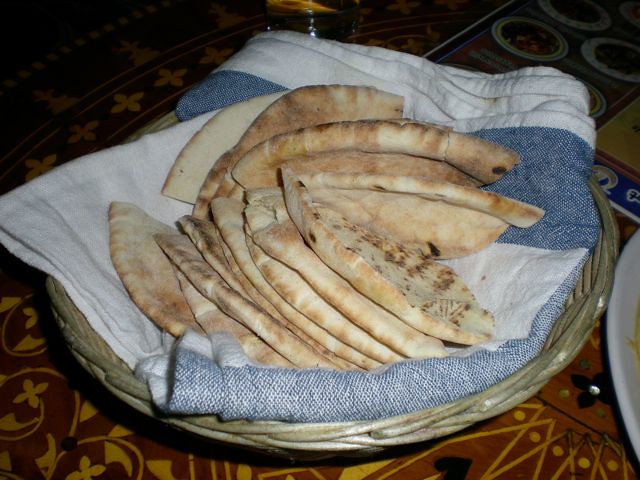This is a detailed color photograph of homemade flatbread, likely Iranian in style but also resembling naan, placed in a greenish-brown wicker basket. The basket is lined with beautifully folded blue and white cloths, enhancing the presentation of the bread. The flatbread, golden with darker spots and cut into triangular pieces, is layered in two distinct piles, one in the front and one in the back, totaling around a dozen pieces. The basket is set against a vibrant backdrop featuring a deep rust and brown tablecloth adorned with lighter graphics, and an orange and yellow patterned surface underneath. A white plate partially enters the frame from the right, and a softly focused menu with circular details appears in the background, suggesting a cozy, inviting dining setting.